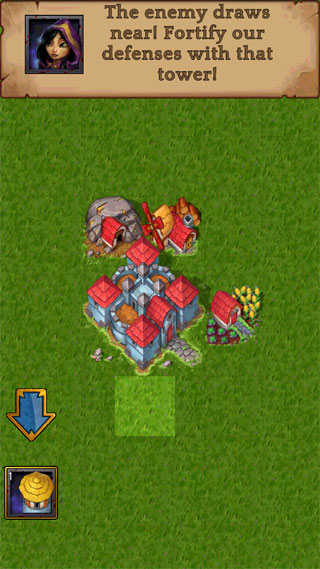This is a detailed screenshot of a mobile game, likely a castle-building type. The aspect ratio suggests it's in portrait mode, similar to a phone screen. At the top of the image, there's a tan-colored text box where a hooded woman is depicted in a small square to the left. She speaks in black text, stating, "The enemy draws near. Fortify our defenses with that tower!" 

Below the text box, the majority of the scene is dominated by a green grassy field. At the center of this field, there is a fortress or castle with distinctive red tiled roofs and grayish-blue walls. Surrounding the central castle are various buildings: one house features a garden, another house appears embedded in rock suggestive of a mine, and yet another house is positioned nearby. Additional details include yellow flowers in front of some buildings and a small square of lighter green grass that seems out of place.

In the lower-left corner of the image, there's a prominent blue arrow pointing downward with a gold outline. Just below this arrow, there's a blue square with a dark blue background. Inside this square is a circular gold object, likely representing a hut or another structure.